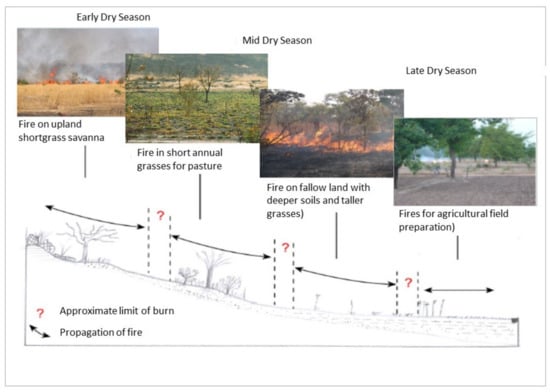The infographic consists of a chart with four photographs illustrating different stages of the dry season in a nature area as it relates to fire management and vegetation. The first photo, labeled "early dry season," shows a fire burning in a field of upland short grass savanna, with additional fires visible in the background. The second photo is marked "mid dry season" and depicts greener land with sparse trees, captioned as being short annual grasses used for pasture. The third image, also labeled "mid dry season," displays another fire, this time on fallow ground with deeper soils and taller grasses. The final photo, "late dry season," features a primarily barren landscape with tall trees and smoke rising in the background, indicating the use of fire for agricultural field preparation. Below these images, a black and white illustration depicts a hillside divided into four sections, each corresponding to the stages and fire management practices shown in the photographs, capturing the cyclical use of wildfires throughout the dry season.